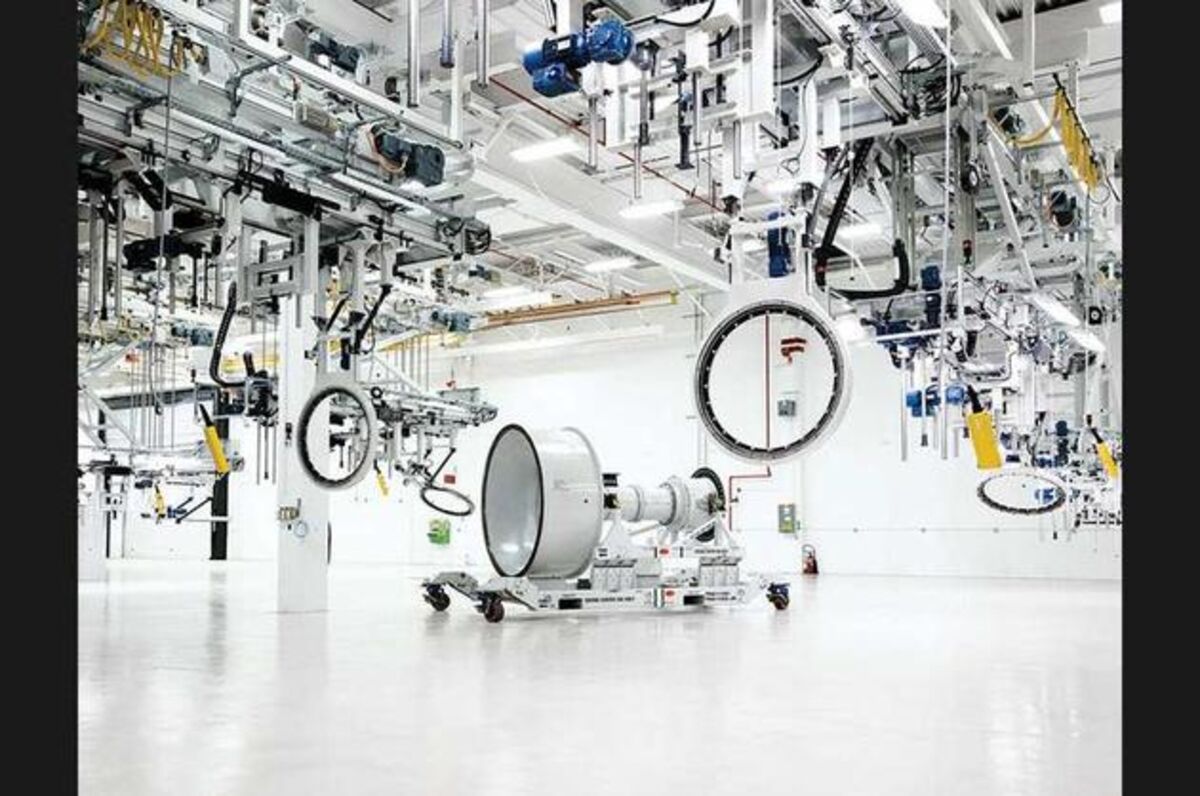This photograph appears to depict an industrial or mechanical laboratory, possibly associated with NASA given the space-related elements described. The scene is dominated by pristine white floors and support columns, creating a clean and sterile environment reminiscent of a hospital. The space is filled with intricate machinery and robotic arms extending from the ceiling, all appearing poised to construct or assemble something complex. The focal point of the image is a large cylindrical object resting on a mobile trolley, suggestive of a rocket part or a significant component of a spacecraft. The equipment and structures are predominantly black, white, and silver, with occasional accents of blue and yellow, adding to the high-tech and monochromatic ambiance. Despite the sophistication of the machinery and the elaborate setup, there are no visible people or identifiable markings, enhancing the enigmatic and futuristic feel of the scene.